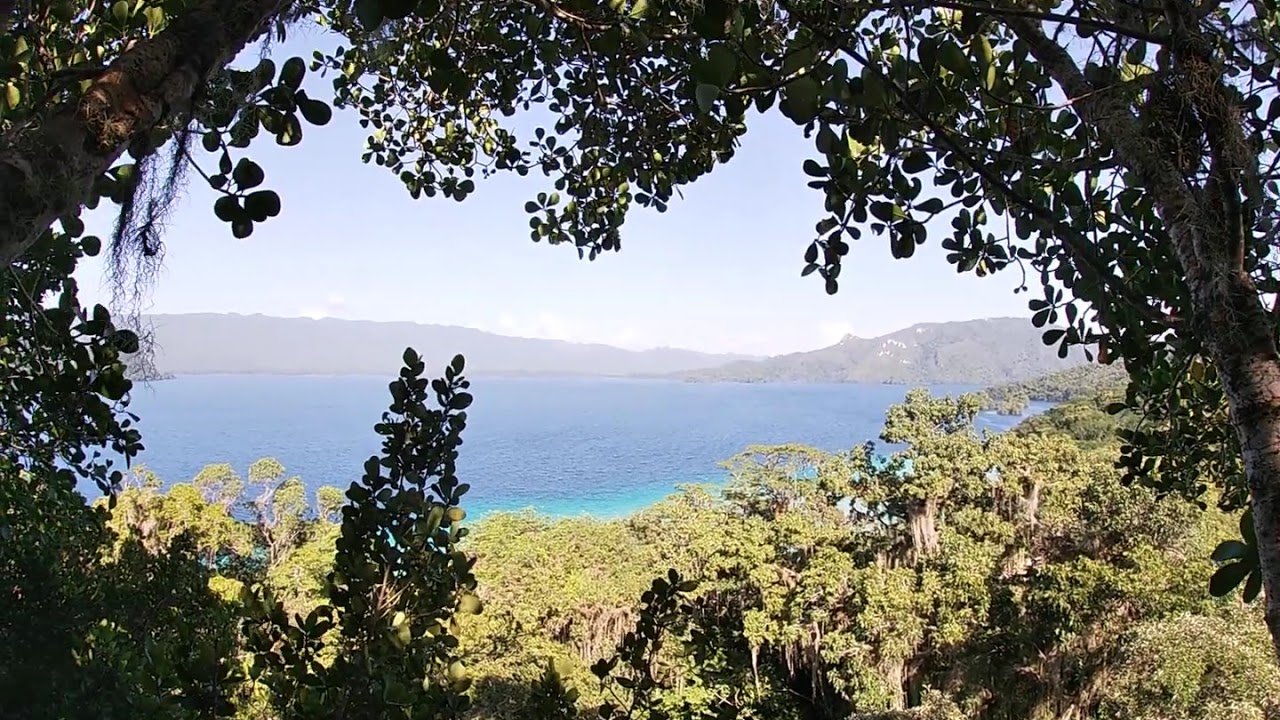The photograph captures a serene outdoor scene on a bright day, taken from a higher elevation. The image is rectangular, approximately six inches wide and three inches tall. Dominating the lower portion is a row of tall, green trees bathed in sunlight. The corners of the photo—lower left, upper left, and upper right—feature overhanging branches and green leaves, creating a natural frame or window through which the central view is seen. This portal-like effect is enhanced by additional green sticks and twigs around the bottom of the frame.

At the core of the image, a striking blue lake stretches from the left center nearly to the right edge, with its near shoreline tinged in a lighter, more teal blue. The surrounding trees on the lake's edge are adorned with green-gray lichen or Spanish moss, suggesting a humid environment. Beyond the lake, low-lying, gray-colored hills or gentle mountains rise up, adding depth to the landscape. Above this, the sky transitions from a near-white at the horizon to a light grayish-blue as it ascends, providing a soft but vivid backdrop to the natural composition.